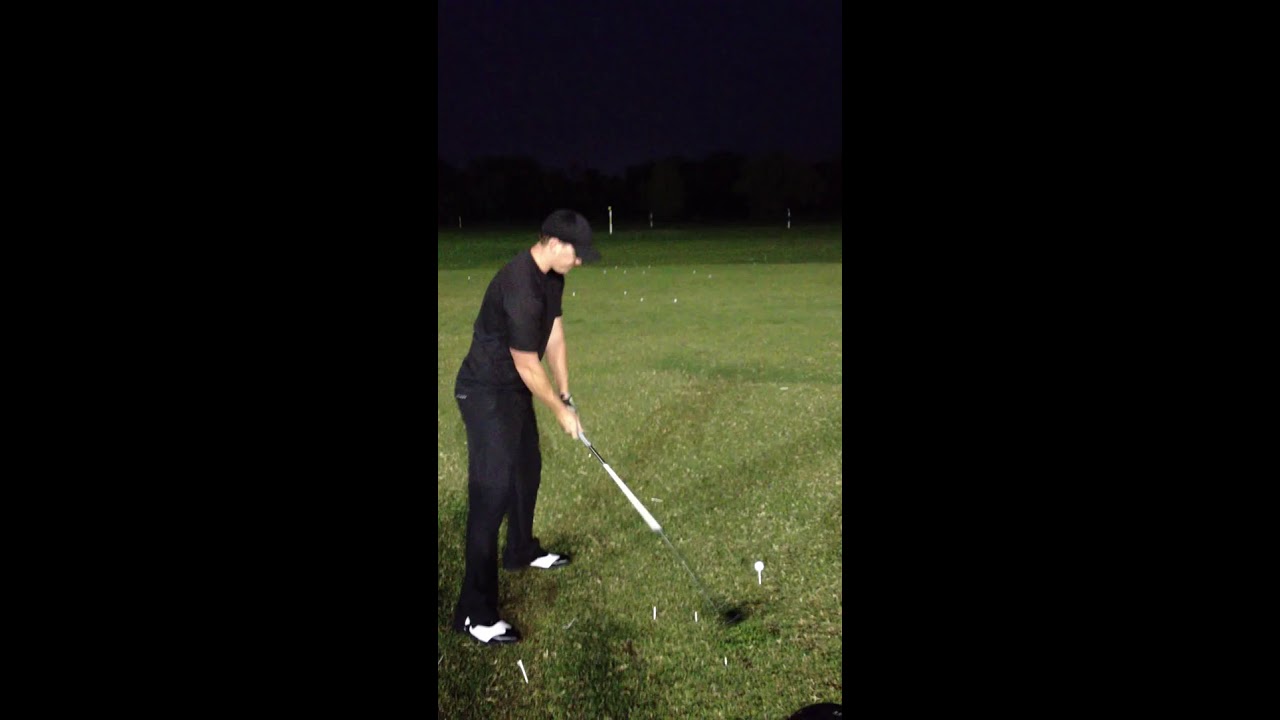In the photograph, a muscular young man is poised for a golf swing at a nighttime driving range. Dressed entirely in black with a t-shirt, pants, and a cap, he stands out against the bright green grass. His black and white golf shoes prominently display their white stripes. The man is preparing to hit a white golf ball placed on a white tee with his golf club, which features a white shaft and grip along with a black head.

The scene is bathed in darkness, with a pitch-black sky overhead and faint silhouettes of trees or hedgerow in the background. Yard markers, distinguishable by their black and white stripes, and scattered white tees dot the green expanse. The image captures the intensity and focus of the golfer amidst the serene nighttime setting.